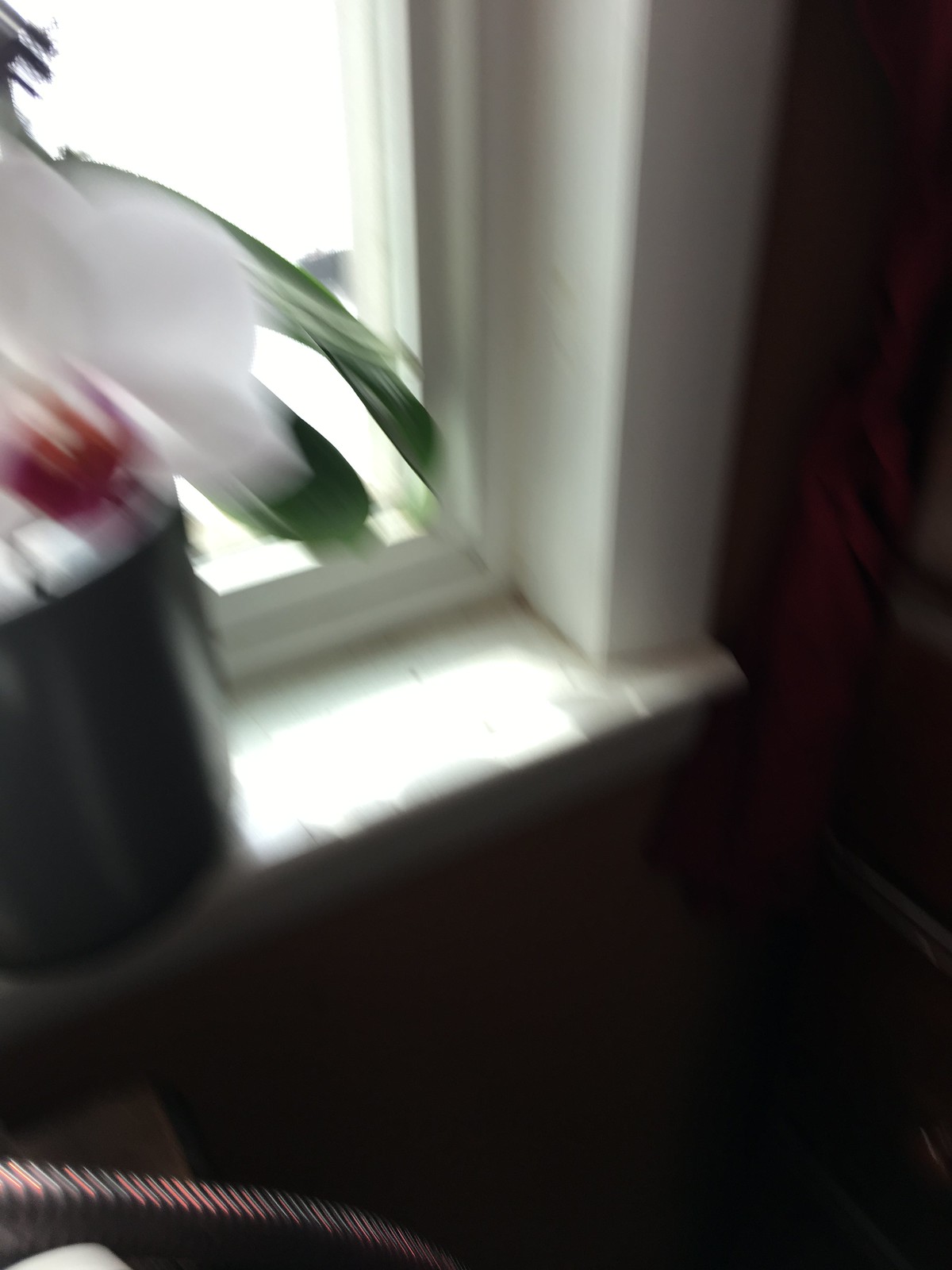A blurry yet captivating image displays a serene windowsill, basking in the soft glow of sunlight that reflects warmly off the white ledge and window frame of the glass window. Perched gracefully on a sleek, black flower pot sits a bird, its delicate neck and vivid plumage illuminated despite the blur. The bird’s body is predominantly white, contrasting beautifully with the vibrant green feathers adorning parts of its tail and wing. Adding to its charm, a touch of black feathers graces the bird's head, creating a striking counterpoint to its lighter hues. The overall scene, though slightly out of focus, exudes a tranquil simplicity that captures a fleeting moment of natural beauty.